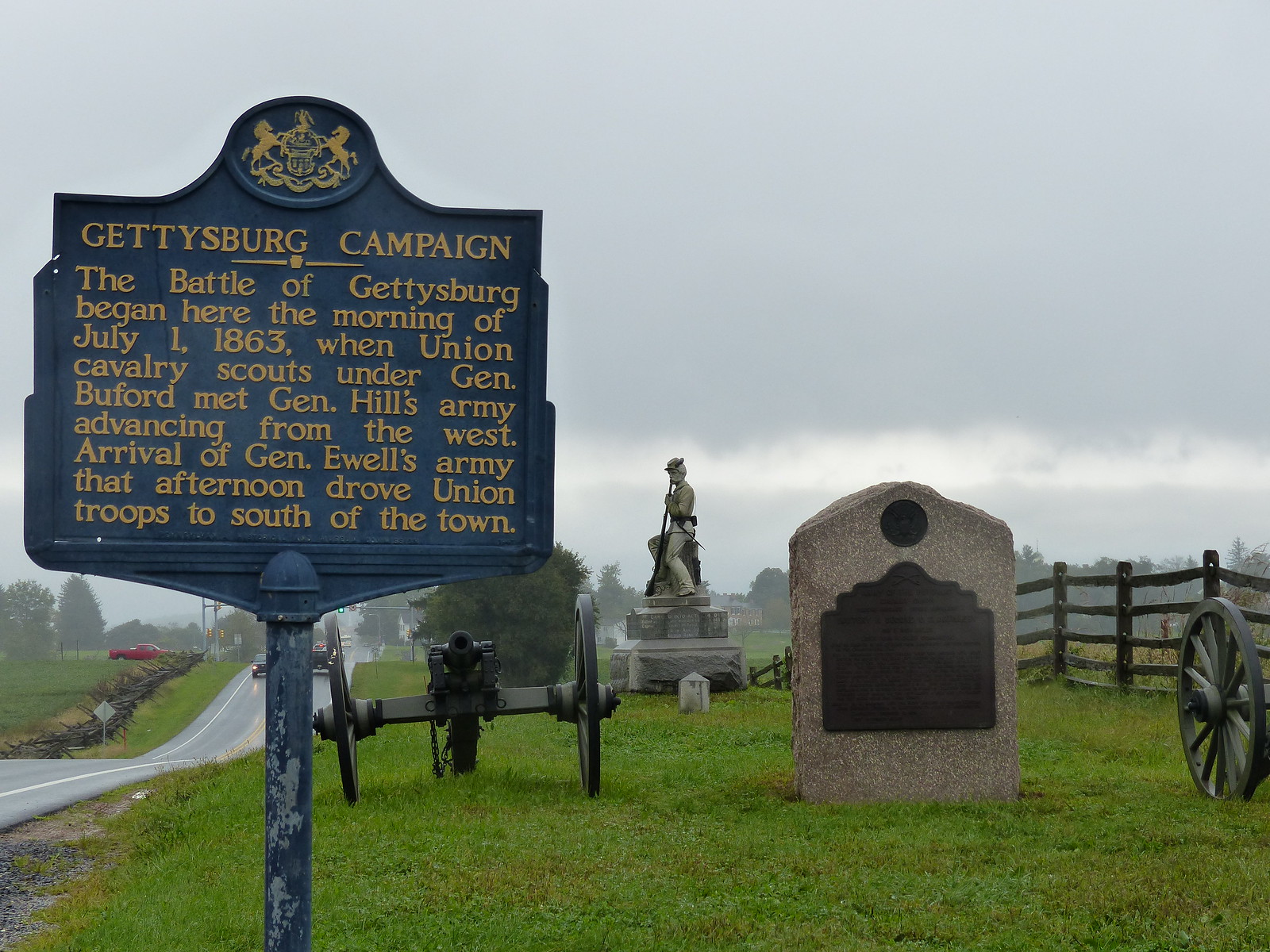The photograph captures a historic monument site on a cloudy, hazy day with a largely gray sky and some white clouds extending horizontally across the middle. This outdoor scene, likely amidst light rain, features a slightly hilly, grassy foreground marked by an old-school cannon on two large wheels facing the viewer. The left side of the image shows a two-lane country road, along which some vehicles are visible with their lights on.

Central to the image is a prominent blue historical marker with yellow lettering, mounted on a worn, brownish-gray metal pole. The sign reads, "Gettysburg Campaign," and provides detailed information about the Battle of Gettysburg, stating, "The Battle of Gettysburg began here the morning of July 1, 1863, when Union cavalry scouts under General Buford met General Hill's army advancing from the west. Arrival of General Ewell's army that afternoon drove Union troops to the south of the town."

To the right of the cannon is a vertical stone monument with an unreadable plaque, and beyond that stands a stone statue of a soldier atop a pedestal, holding a rifle. A second cannon is visible to the far right, and a wooden picket fence stretches across the field, suggesting the area is part of a historic battlefield, likely the site where the Battle of Gettysburg commenced.